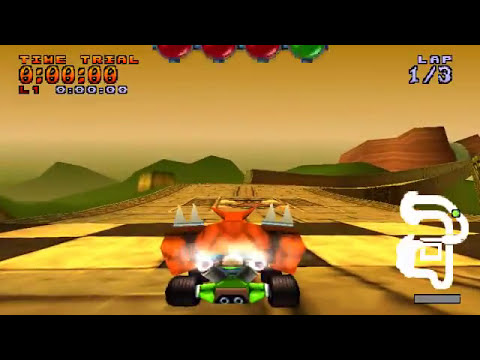This is a horizontally rectangular still image from a racing video game, accentuated by black borders on the top and bottom. The main feature is a vibrant scene set on a wide, golden-brown road in a mountainous landscape. The background displays green and brown mountains shrouded in green fog, with a sky that transitions from yellow to grayish-yellow. Central to the image is a green race car with bright red highlights, four small black wheels, and four metallic gray spikes on its top. The car, emitting red flames, hints at high speed and readiness to race. In the upper left corner, orange text reads "Time Trial, Level 1" followed by zeros, indicating no elapsed time. Below this, white zeros add further emphasis. To the right, at the upper edge, are three red balls and one green ball, while the upper right corner states "Lap 1 of 3." The lower right corner features a green dot representing the car’s location on a racetrack map.